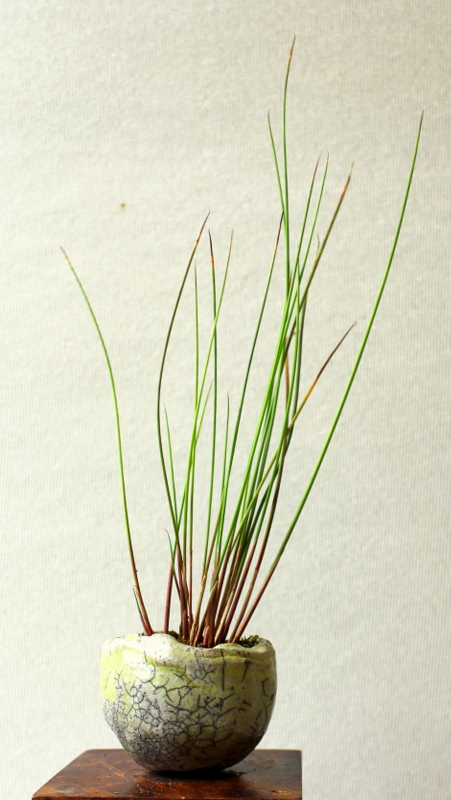The photograph features a potted plant on a small, worn wooden side table. The backdrop of the image is a canvas-like gray fabric wall, with visible ridges and textures that suggest a material with depth and character. The plant resides in a ceramic or clay pot, intentionally designed to appear aged with deliberate gray cracks. The pot itself is an ivory-white color, adorned with sporadic yellow spots, resembling a dinosaur egg cut in half. Emerging from this unique planter are multiple long blades of grass, green towards the edges and top but transitioning to brown as they near the pot. The photograph, taller than it is wide, captures the striking contrast between the verdant grass and the aged, textured pot, presenting an almost museum-like piece of botanical art.